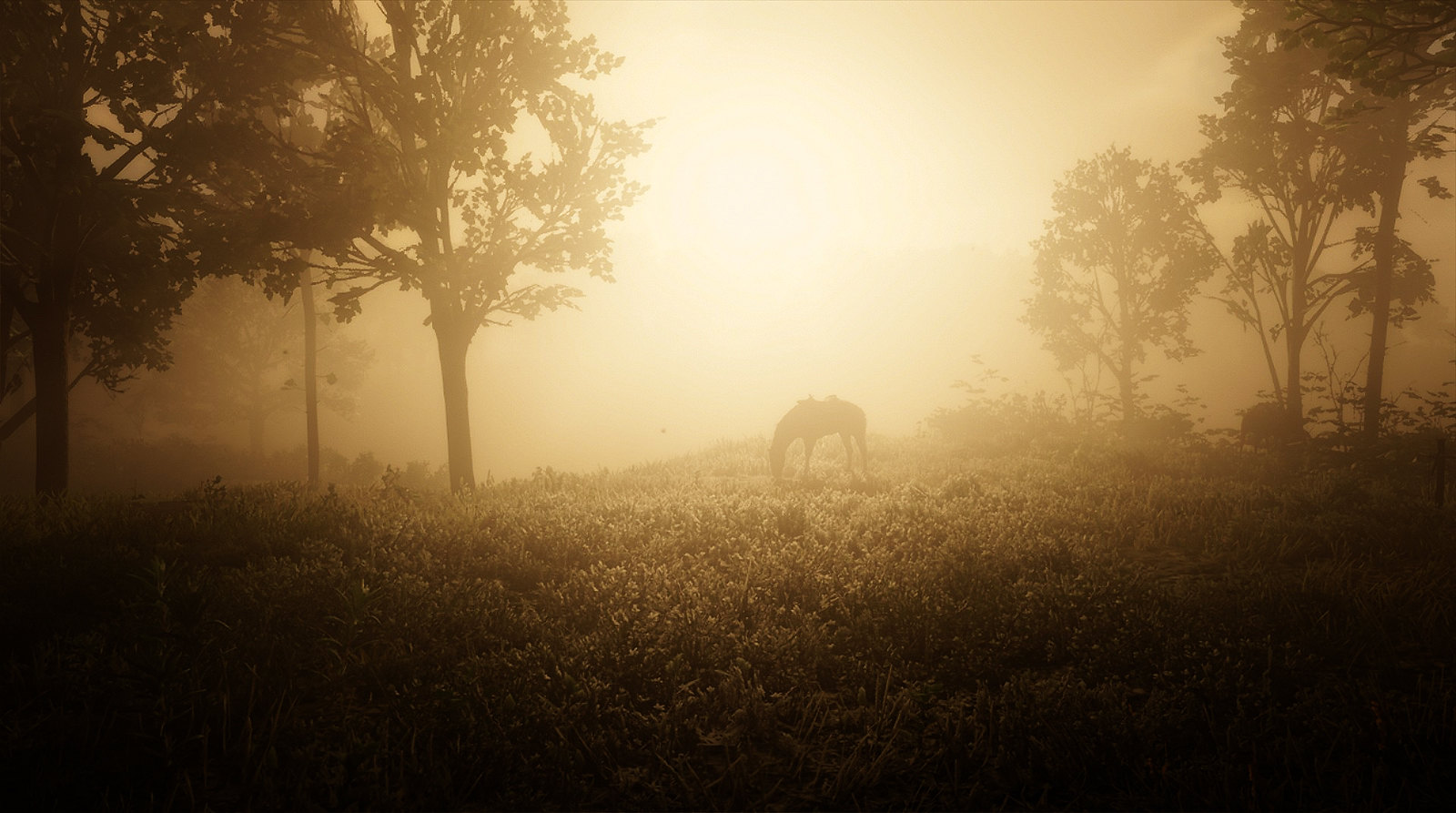In this serene, almost monochromatic photograph, a gentle light brown tint permeates the entire scene, casting a warm, nostalgic glow. The sky, slightly hazy with a muted brown hue, softly filters the late afternoon sunlight. Below, a vast pasture stretches out, its rich expanse of grass punctuated by clusters of bushes and robust, sprawling trees. At the center of this tranquil landscape stands a solitary horse, peacefully grazing, its figure a harmonious part of the pastoral setting. The corners of the image are enveloped in deep shadows, adding to the overall somber yet peaceful ambiance, making the scene feel both timeless and secluded.